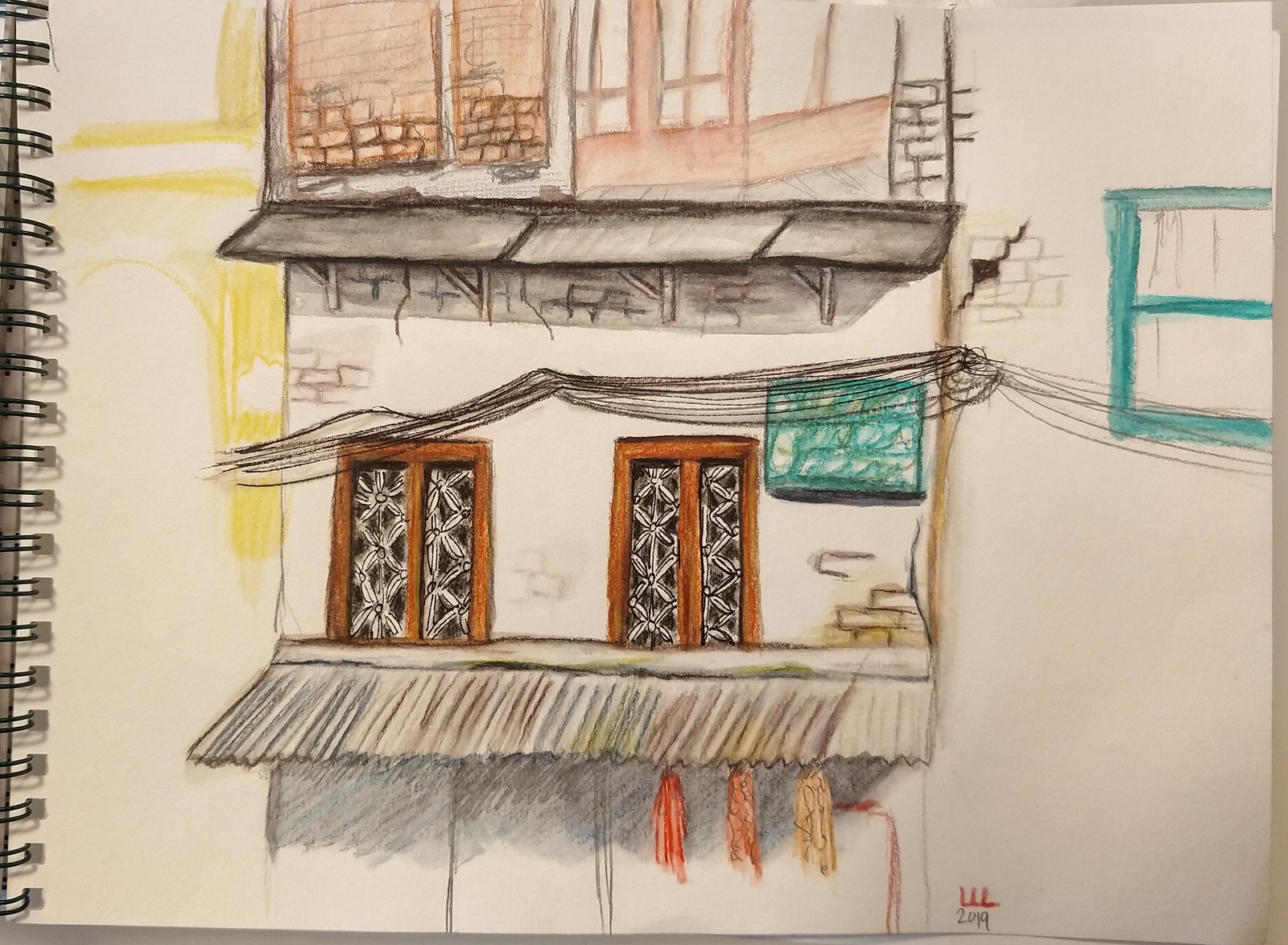This is a detailed, colored pencil drawing captured within a white spiral-bound sketchbook. The book is held together by black rings along the left edge. The image depicts a multi-story building, possibly a typical house in the Philippines, featuring distinct architectural elements. The building showcases a sheet metal roofing designed to catch rain, with various canopies shading the structure. The second story displays two tall, rectangular windows framed in brown, while adjacent, there is a separate, teal-framed window. The illustration highlights red shutters, some featuring black interiors, and intricate window details suggesting stained glass patterns. Bricks are artistically shaded in different areas, adding to the texture, with a mix of colors including yellow, green, red, gray, and brown. The drawing is annotated with "2019" at the bottom, possibly accompanied by an indecipherable name. The background surface, partially visible on the right, appears smooth and gray.